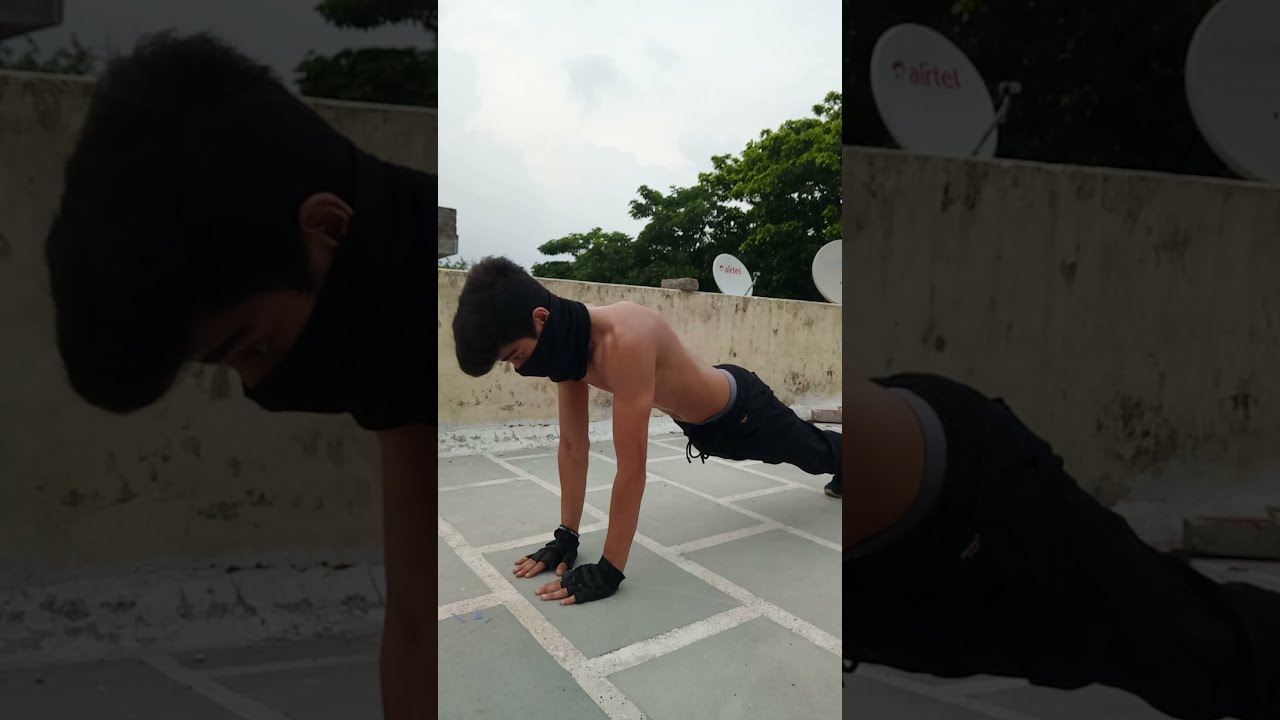The image depicts a shirtless young man, likely Asian and in his late teens or early 20s, poised in a push-up position on a rooftop patio. He has a distinctive hairstyle with long black hair on top and short sides, including sideburns. His facial features are partially obscured by a mask or scarf covering his mouth and nose. He wears black workout gloves with the fingers exposed, black sweatpants, and black tennis shoes.

The rooftop patio features rectangular gray stone tiles with contrasting red grout lines, and a concrete wall behind him. The wall, slightly brownish or reddish white, angles towards the right. Above the wall, there are two white satellite dishes marked "Airtel," and green tree leaves are visible against a whitish-blue cloudy sky. Additionally, the image has magnified, grayed-out sections on both the left and right edges: the left section focuses on his face and one arm, while the right section highlights his midsection, pants, and part of the wall and satellite dishes.